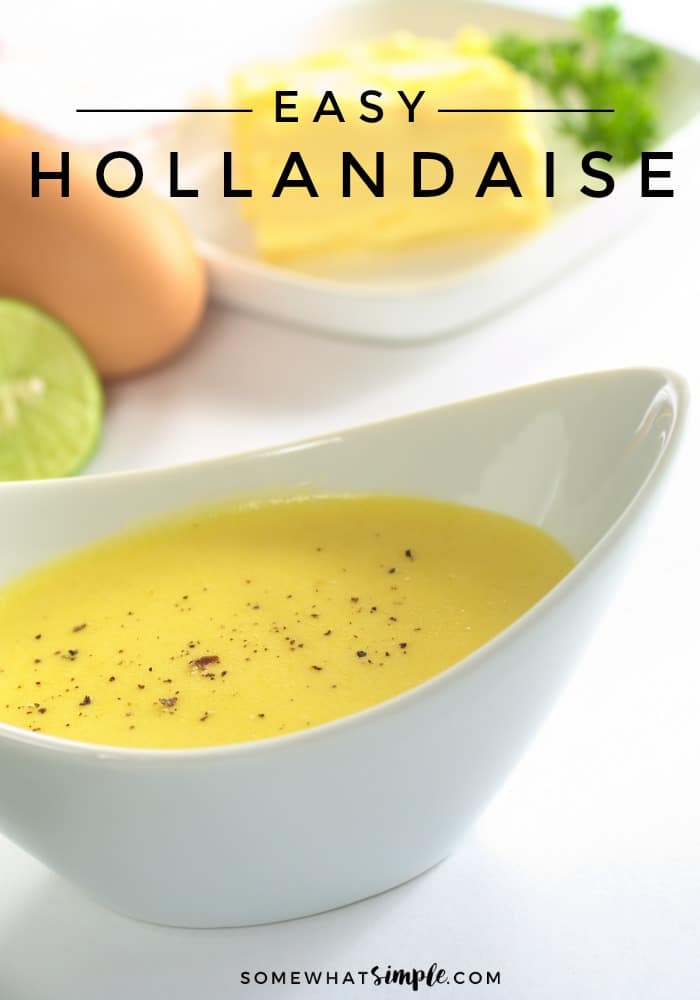The image prominently features a white, reflective bowl filled with yellow Hollandaise sauce, sprinkled with pepper or herbs, positioned slightly to the left in the forefront. Above the bowl, the text "Easy Hollandaise" is displayed in black letters. In the background, there's a butter dish containing butter, a sprig of parsley or green leaves, an egg, and a sliced lime, slightly blurred. The bottom of the image features the text "SomewhatSimple.com" in black over a white table surface. The overall feel of the image is clean and emphasizes a simple, homemade presentation of the Hollandaise sauce.